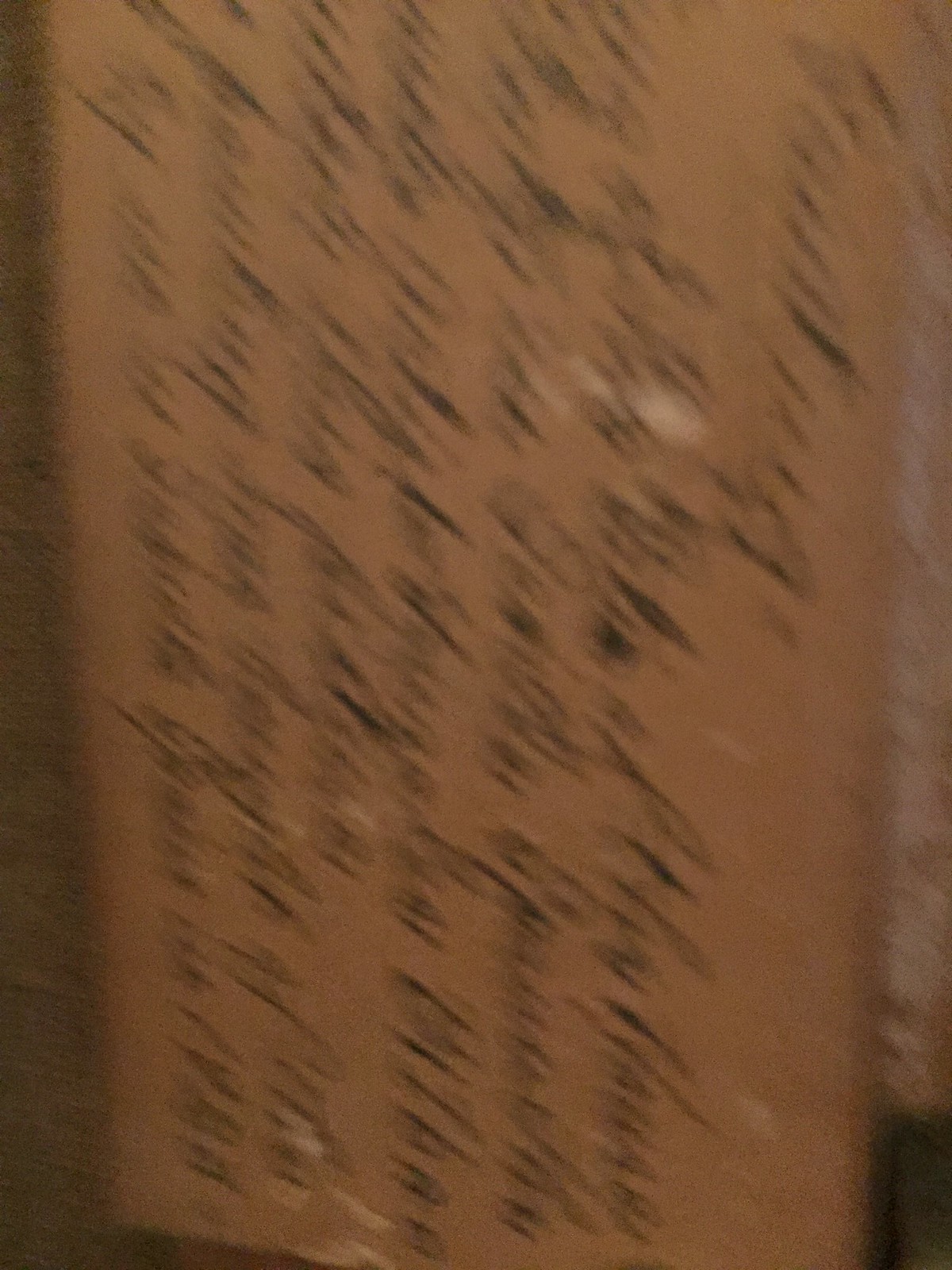This image features a blurry photograph of a small, aged piece of paper, likely oxidized, giving it a brownish hue. The paper contains cursive handwriting, reminiscent of the elegant script produced by old ink pens predating the ballpoint era. The ink appears uneven, with noticeable heavier droplets, suggesting the use of a traditional fountain pen. Despite the blurriness obscuring the content, the script exudes a historical charm, indicating that it could potentially be an old note, recipe, or some other handwritten document. The size of the paper is relatively small, emphasizing its delicate and perhaps intimate nature.